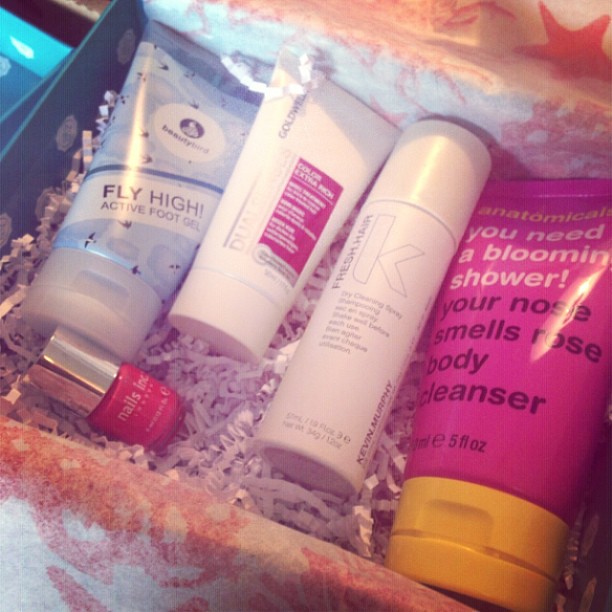The image shows a beauty box of personal care products set against a decorative coral, beige, and white floral or leaf-patterned box with white crinkle-cut packing strips inside. On the left, there's a bluish tube with a clear lid labeled "Fly High Active Foot Gel," featuring a circular logo at the top. To its right, a white tube bears a red square, with the word 'color' partially readable. Continuing right, there's a light brownish beige cylindrical bottle identified as "Fresh Hair K" by Kevin Murphy. Next is a pink squeeze bottle with a yellow-orange cap, branded "You Need a Bloomin' Shower. Your Nose Smells Rose Body Cleanser." Finally, at the bottom left corner of the box lies a small red nail polish bottle with a gold-tinted clear cap. The entire box is illuminated with natural daylight, which enhances the visibility of the items.